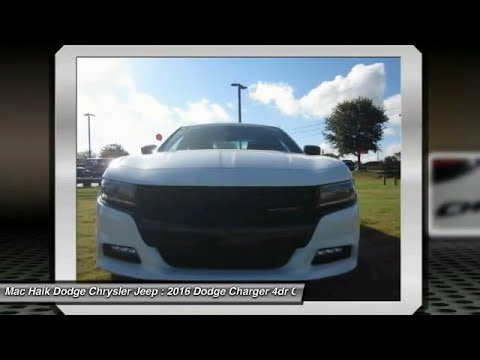The image is a detailed, frontal photograph of a white 2016 Dodge Charger 4DR, prominently displayed within a white-bordered frame resembling a slide from a slideshow. The border itself is part of a larger still, with another out-of-focus frame visible to the right. Outside the frame, there's a gray box with a black border, featuring the text "Mack Hike Dodge Chrysler Jeep: 2016 Dodge Charger 4DR" in white font. The top and bottom of the image are flanked by vertical black bars, with the top one obscured by the shading of the upper screen. The bottom of the screen reveals a grid-like texture. The car is parked on green grass beneath a blue sky with clouds, and a tree is on the right side. Light poles are also visible in the background, indicative of the car being in a park-like setting. The car's headlights, grill, and windshield are clearly visible, dominating the center of the composition. This setup suggests the image could be part of an advertisement or a presentation slide promoting the vehicle for sale.